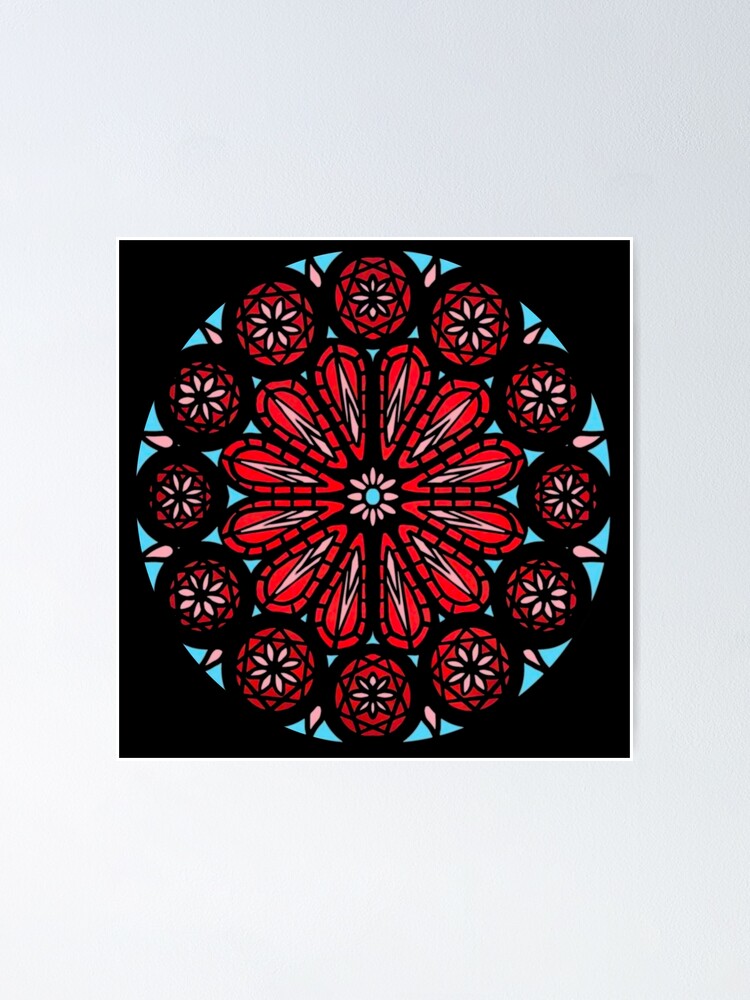The image depicts a detailed illustration of a stained glass window, rather than an actual photograph of one, set against a gray background. The design's symmetrical composition features a central red section adorned with a flower pattern. Surrounding this central motif are about 12 to 14 medallions or circular shapes, each containing floral designs, highlighted in white and bordered in black. These medallions form a larger circle around the center. The entire artwork is bordered in black. Behind the intricate patterned circles and flowers, a light blue color fills the space, enhancing the vivid red and white contrasts within the intricate floral designs. The illustration is meticulously detailed, possibly created digitally, highlighting its ornamental and geometric aesthetic devoid of any religious symbolism.